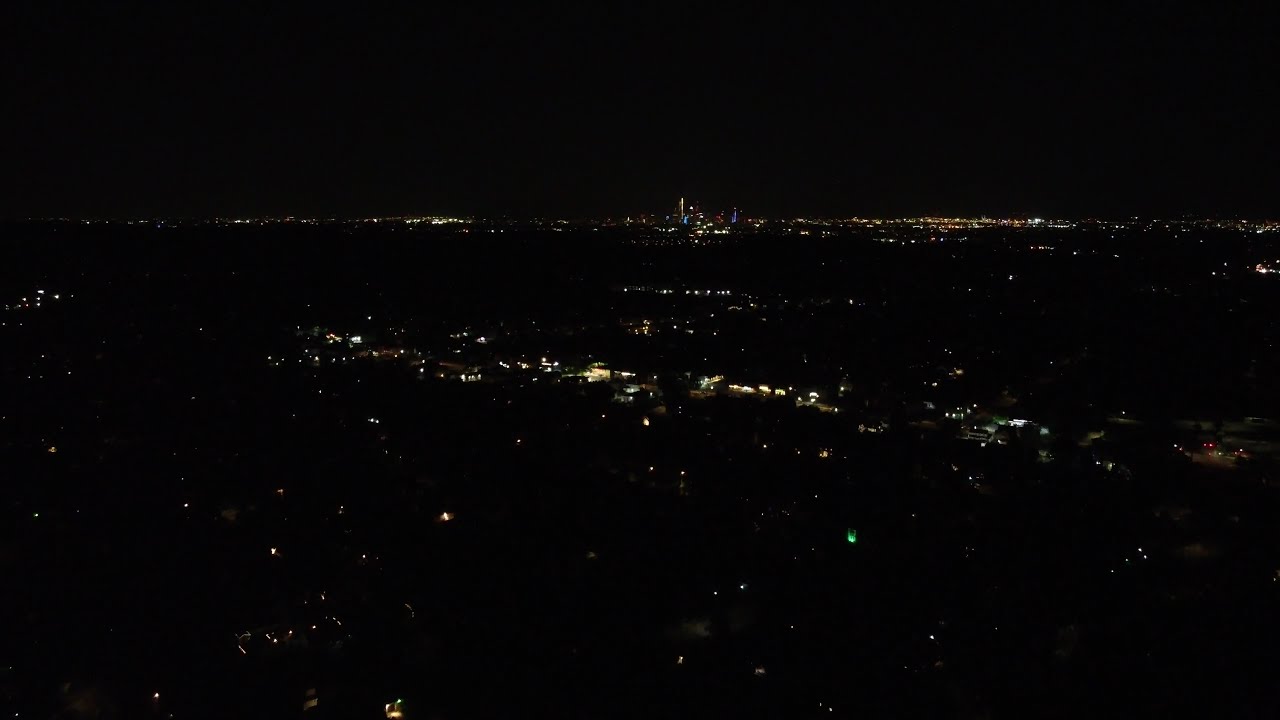The image depicts an aerial view of a cityscape at night. The photograph captures a predominantly dark and almost pitch-black sky devoid of stars. The horizon features a long row of golden and white lights that outline a distant city with several tall skyscrapers. In the middle of these structures, one skyscraper glows with a purple hue to the left and another emits a blue light to the right, while others display a variety of lights including white. Throughout the image, scattered lights of different colors, namely black, white, yellow, blue, and red, illustrate the positions of various buildings, both residential and commercial, dotting the landscape. Toward the bottom of the image, a glowing road runs horizontally, marked by a mix of amber and white lights trailing along its path. The overall setting is a very dark night scene characterized by scattered illumination, making the specific details of the buildings hard to distinguish.